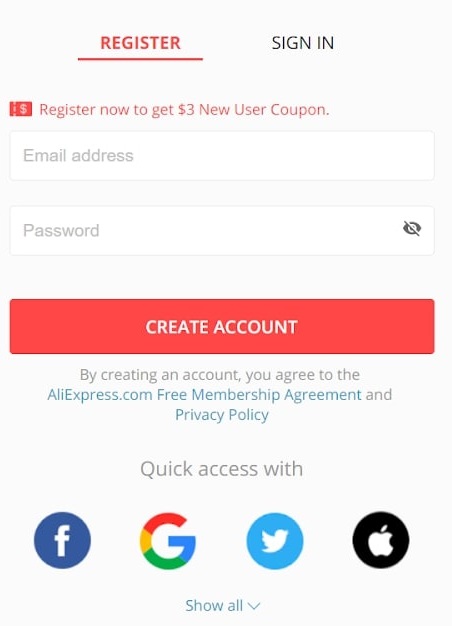The image depicts a registration page for AliExpress with detailed instructions and options for creating a new account. At the top, there's a prompt encouraging new users to sign up to receive a $3 coupon. Below this, the page features input fields for entering an email address and password required for registration. There is also a CAPTCHA verification component described as "some kind of I."

Prominently displayed is a large red rectangle button with white text in the center that says "Create Account." Beneath this button, there is a disclaimer stating, "By creating an account, you agree to the AliExpress.com Free Membership Agreement and Privacy Policy."

The image also includes several quick access buttons for alternative registration methods via social media accounts. These include a blue circle with an "f" for Facebook, a multicolored "G" for Google, a blue bird for Twitter, and a black circle with an apple logo for Apple ID. Each icon is vividly colored, with the Google "G" notably including red, yellow, green, and blue segments.

The final text at the bottom re-emphasizes the process to register on AliExpress.